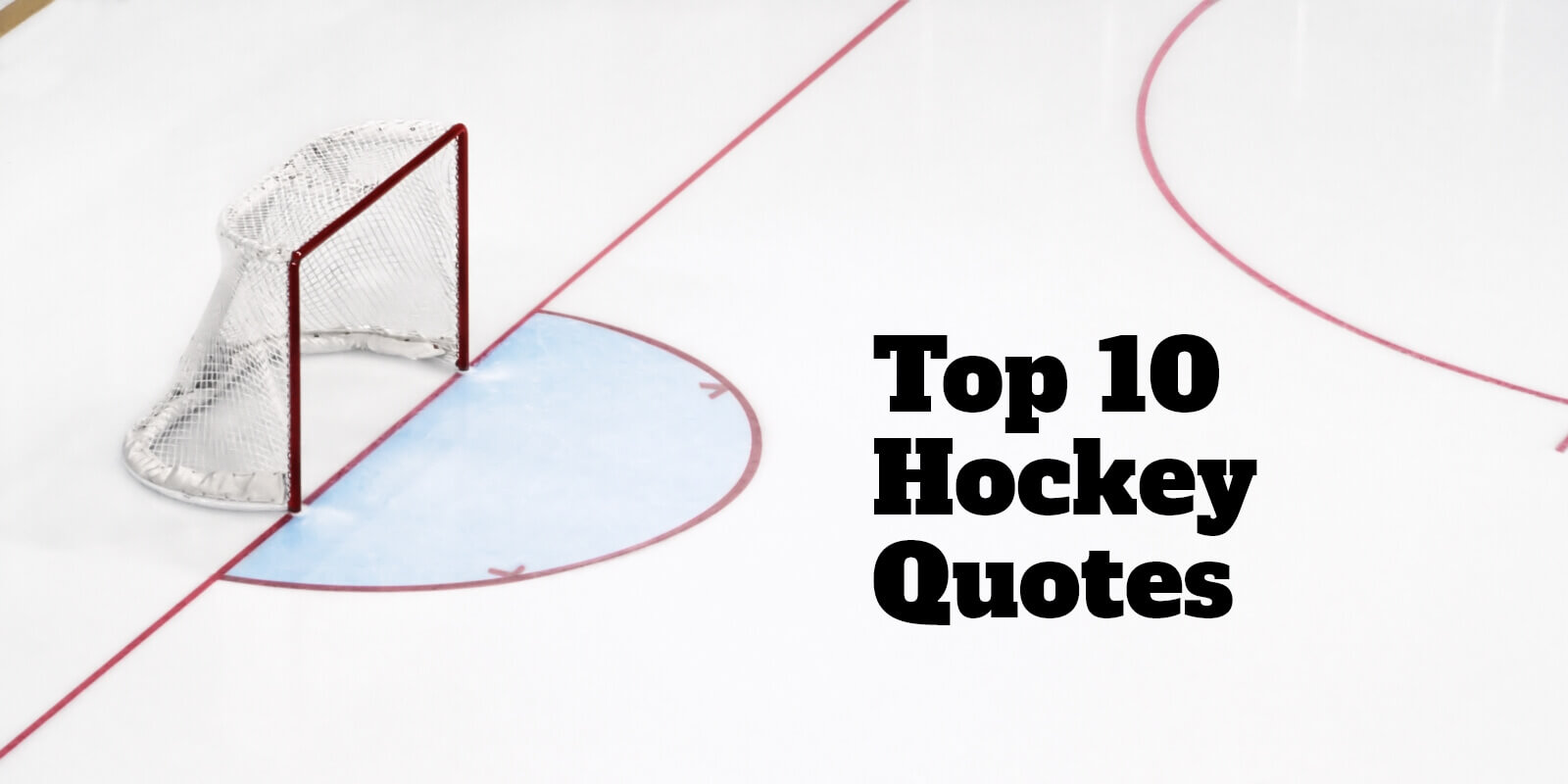The image depicts a graphic representation of a hockey arena, with a focus on one of the goals positioned on the left side. The goal features a net with a red goal line running in front of it, and a surrounding blue semicircle outlined in red, indicating the goalie's area. To the upper right of the image is part of another red circle, commonly used for face-offs. The background is white, symbolizing the ice rink. Central to the image, in bold black text, appear the words "Top 10 Hockey Quotes" written in title case. This text is positioned between the two red circles, approximately halfway down from the top.